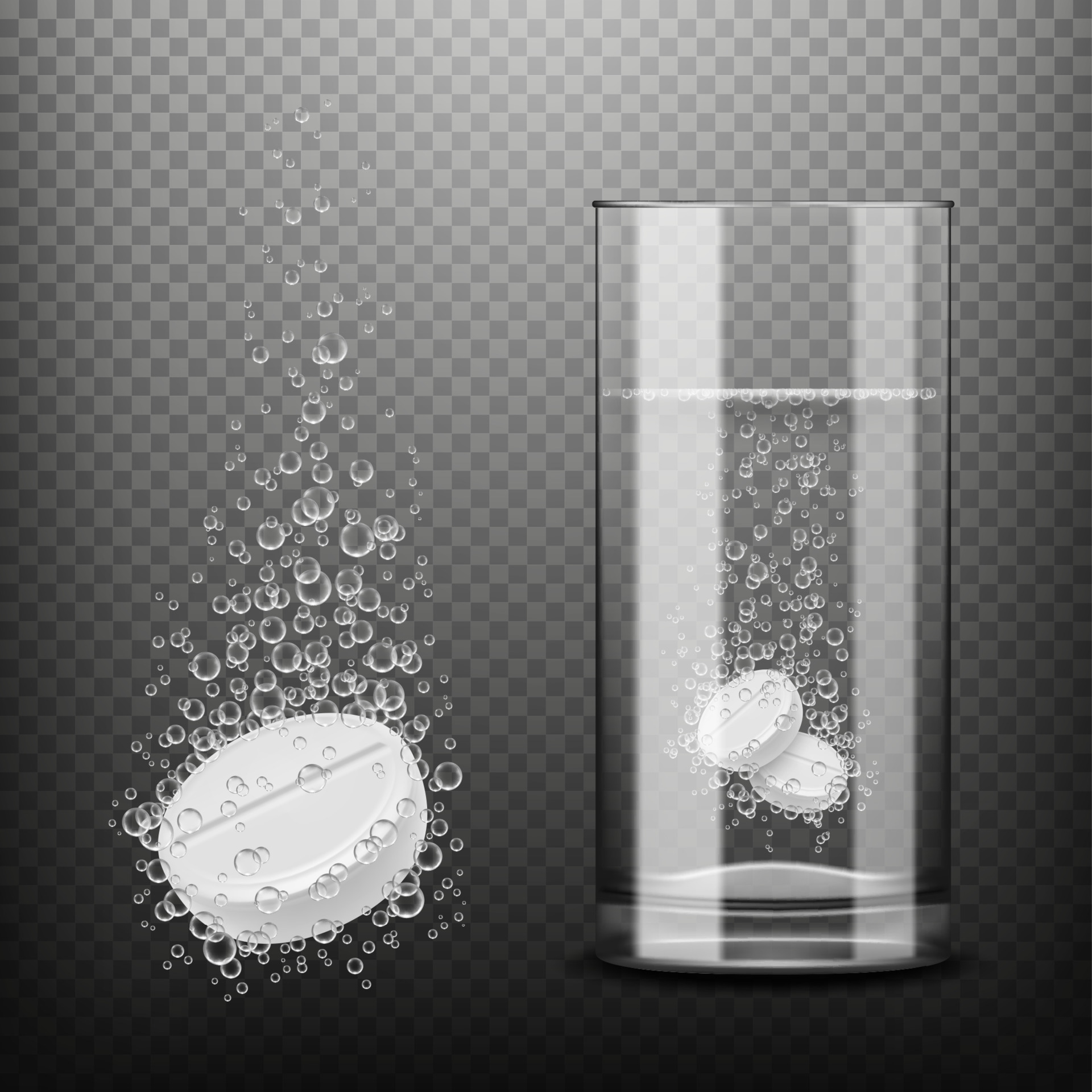In this detailed black and white image, a single white, round Alka-Seltzer pill with a line bisecting its center is positioned on the left. Bubbles radiate from the pill, giving a sense of effervescence. Adjacent to this pill, on the right side of the image, stands a tall cylindrical glass filled about three-fourths with water. Within the glass, two similar white Alka-Seltzer tablets, also with central lines, rest at the bottom, releasing a cascade of bubbles that rise to the surface. The background features a checkered pattern with varying shades of gray, from light at the top to darker hues at the bottom, creating a gradient effect. The glass captures and reflects some light, adding a subtle layer of complexity to the scene. This image seems to evoke a sense of action characteristic of an advertisement or promotional clip art for the fizzing medication.